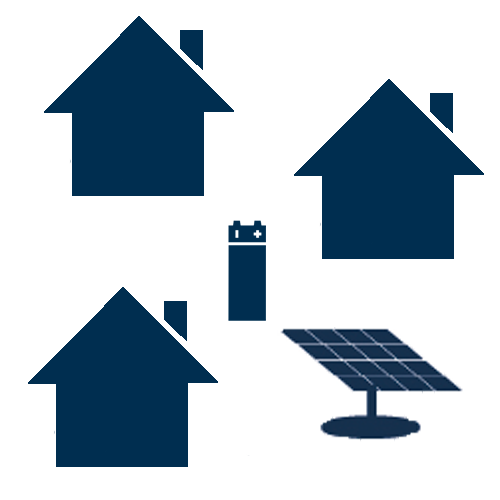The image features a minimalist, iconographic illustration on a pure white background. In the top left (quadrant 1), top right (quadrant 2), and bottom left (quadrant 3) corners, there are three identical dark blue house icons. Each house has a square base, triangular roof, and a simple rectangular chimney on the right side of the roof. Notably, the house in the top right corner is positioned slightly lower than the one in the top left corner, by approximately 5%. In the very center of the image, there's a 9-volt battery icon with two bumps on top, marked by a plus sign on the right and a minus sign on the left. In the bottom right corner (quadrant 4) is a solar panel icon, which features a dark blue base and a cylindrical stand that supports a 4x4 grid of panels angled towards the upper right. All these elements are uniformly styled with simple, shaded-in shapes, emphasizing their symbolic nature.